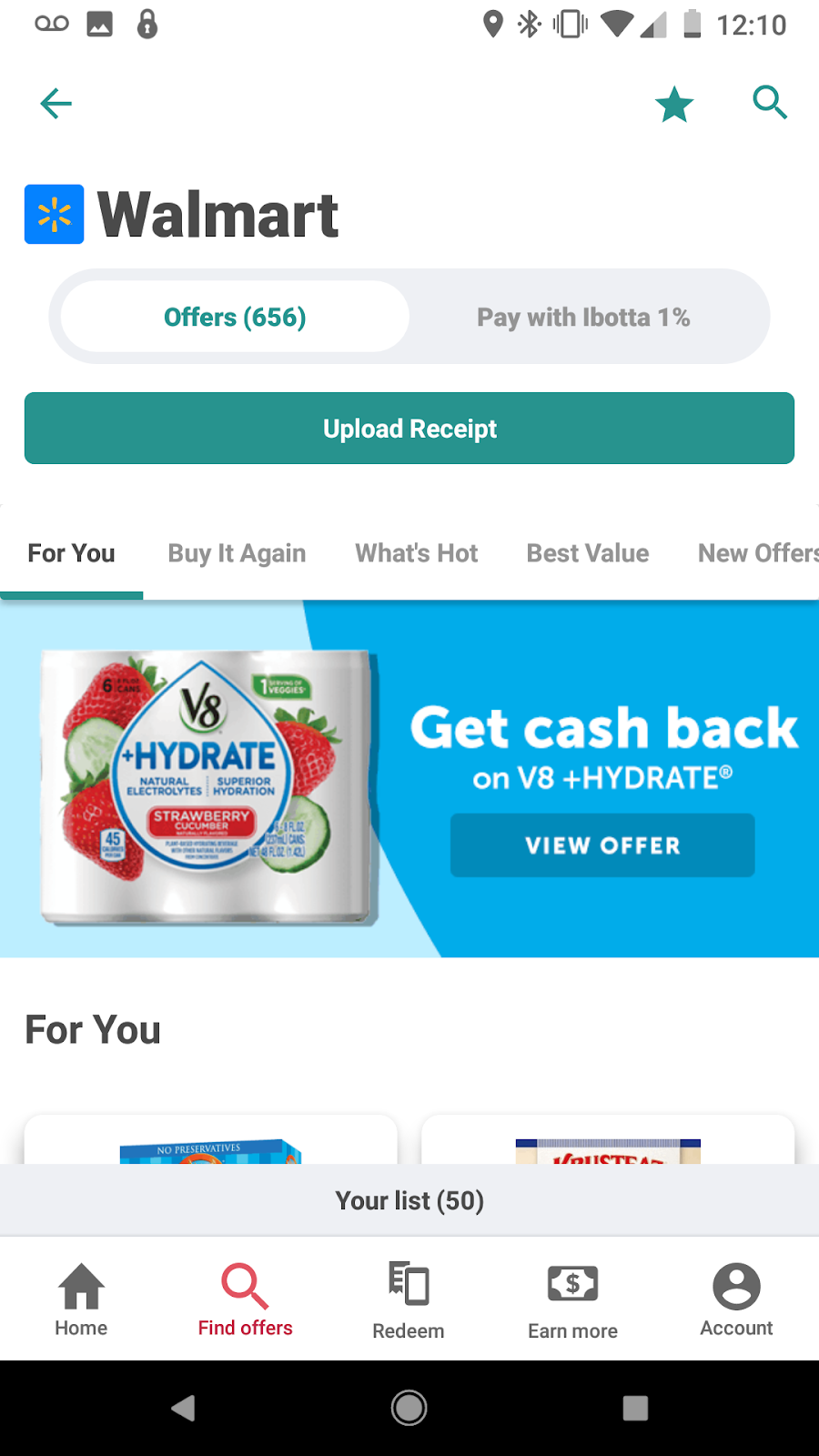The screenshot captured on a smartphone at 12:10 PM with a nearly empty battery (10-20% remaining) is from the Ibotta app, showing the Walmart section. The upper left corner displays the Walmart logo, characterized by a yellow firework design inside a blue square. Directly beneath the logo, the screen lists "Offers" with a total of "656 offers" noted in parentheses. To the right, the option to "Pay with Ibotta" is visible, indicating the app’s functionality for scanning receipts and availing cashback offers. A prominent green "Upload Receipt" button is also displayed. Beneath this, the navigation bar shows multiple options with "For You," highlighted by a green underline, currently selected. An offer to "Get cashback on V8 + Hydrate" with a clickable "View Offer" button is prominently featured.